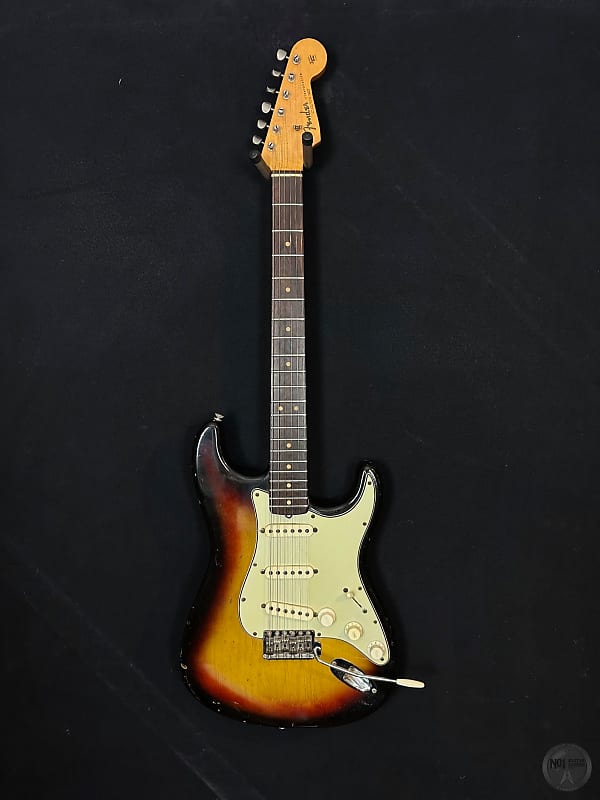This is a detailed close-up photograph of a Fender electric guitar against a completely black background. The guitar, which appears to be hanging on a wall, features a sunburst finish with shades of burnt orange and yellow on its body, transitioning to darker edges that are almost black or dark brown. The wooden neck is light brown, and the headstock, which holds six white tuning knobs, is supported by a hook. The instrument includes a whammy bar, metal strings, and three fine-tuning knobs alongside one slider on its body. The bottom right corner of the image showcases a circular watermark, which is partially obscured but seems to say "NOI" followed by additional text. The guitar is resting on a dark gray, velvety cloth, and the photograph is taken in portrait mode, emphasizing the guitar's vintage and well-loved appearance.